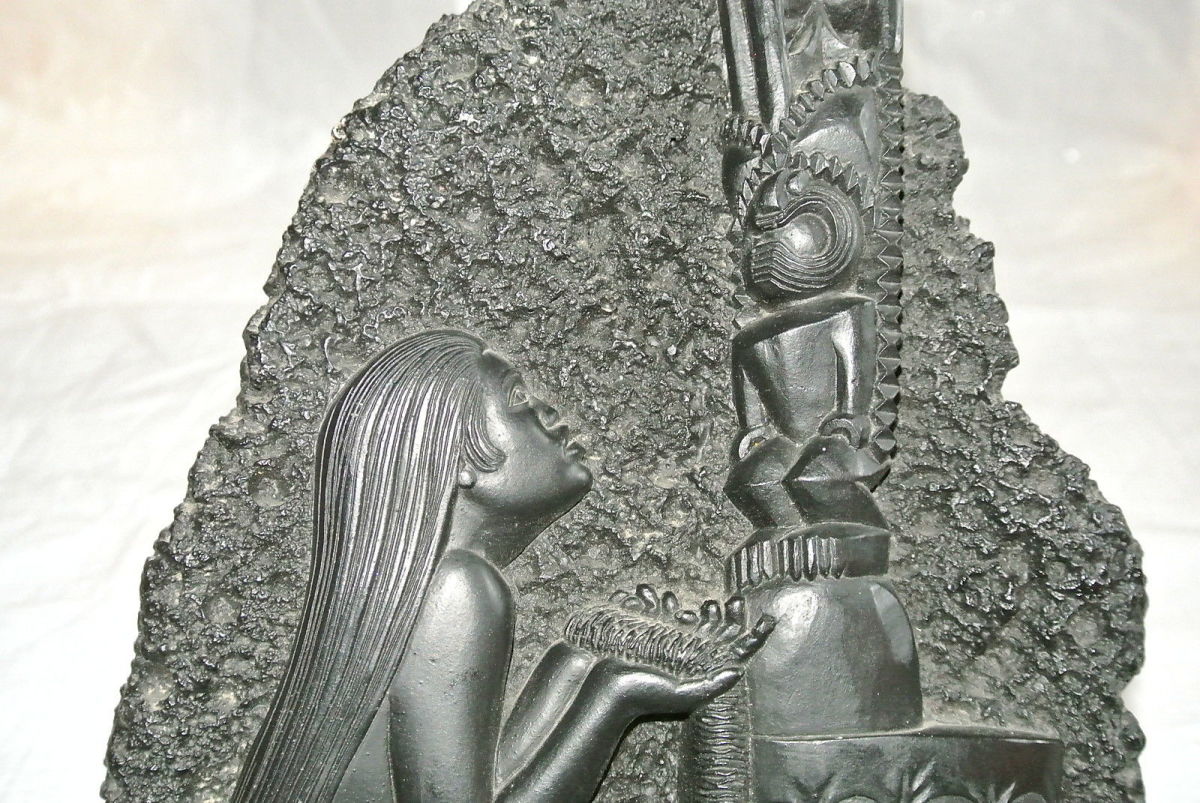This is a detailed photograph of a carved sculpture made from crinkly, textured lava rock, prominently featuring a triangular overall shape with a dark grey and somewhat shiny surface. The central figures in this artwork are zoomed in, cropping out the broader context but highlighting intricate details. To the left of the sculpture, there is a side profile of a kneeling Polynesian woman with long, straight hair cascading down her back. Her hands are raised, palms up, as if offering something to a figure beside her. On the right, standing on top of some stones, there is a Tiki God totem extending from the bottom to the top of the image. This Tiki God appears humanoid yet animalistic, with disproportionate arms and legs, and bears a face adorned with geometric designs akin to a mask. The background behind these figures is roughly chiseled to contrast with the smoother look of the carved subjects, and the edges of the sculpture show signs of wear or breakage, resting on some kind of white fabric.